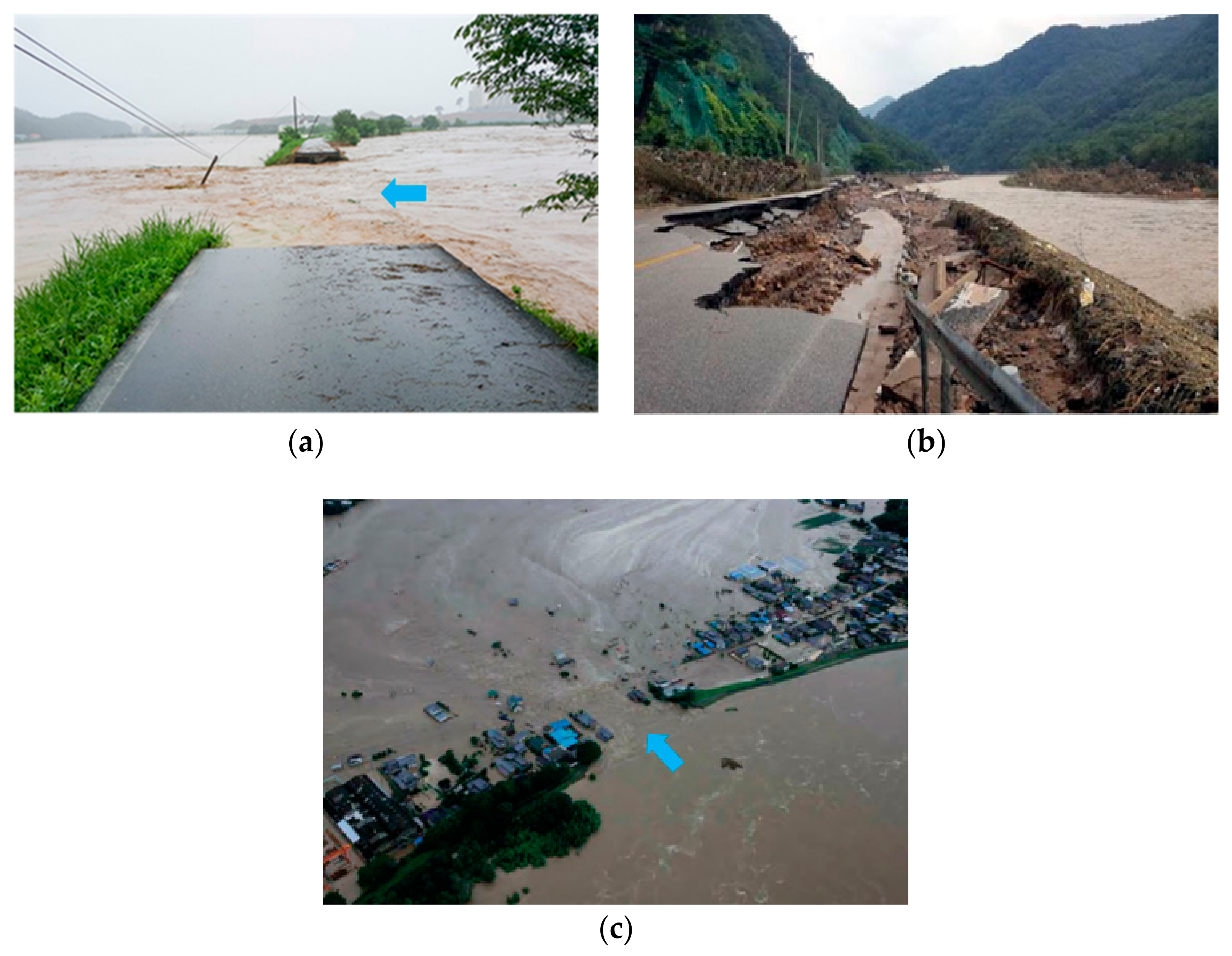This composite image consists of three separate photos labeled A, B, and C, showcasing the devastating effects of severe flooding.

**Image A (Top Left):**
A paved road has been partially destroyed by a surge of muddy brown water cutting horizontally across it, illustrating the immense power and chaos of the flood. Power lines are visible in the background, with one pole almost completely submerged in the water, emphasizing the severity of the flooding. A blue arrow marks the exact location where the road has been washed away.

**Image B (Top Right):**
This image captures a roadway running adjacent to a mountain on the left and a river on the right. The road is visibly crumbling and deteriorating, succumbed to the floodwaters. Another mountain looms in the distance on the right. The image highlights the precariousness of infrastructure in the face of natural disasters.

**Image C (Bottom):**
A parking lot is shown in a grid-like arrangement, now engulfed by floodwaters. Cars are parked in neat rows, but water has invaded the entire area, turning it into a miniature lake. A blue arrow indicates the specific area where water is flowing through and causing the inundation.

Each image powerfully depicts the destructive force of flooding, from washed-out roads to submerged infrastructure.